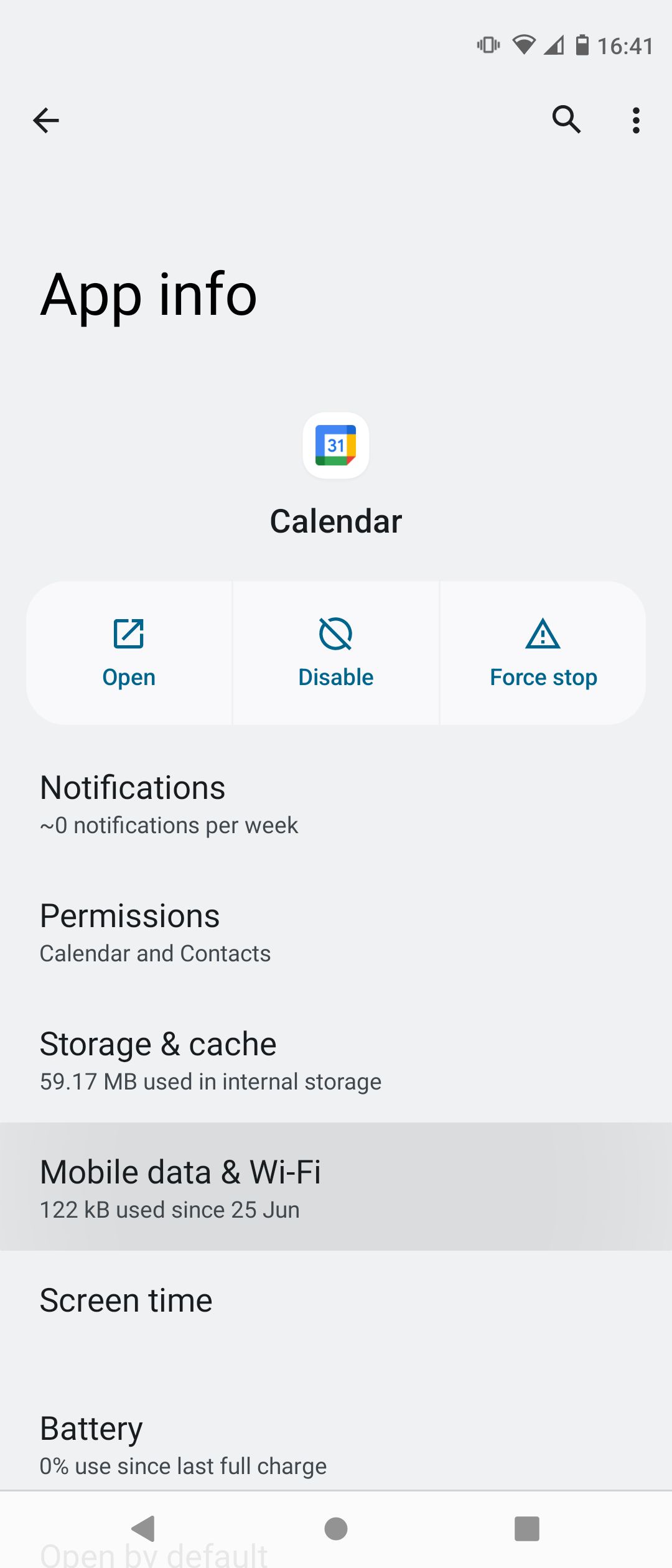This digital image is a screenshot taken at 16:41 (military time) showcasing detailed app information. The interface displays a prominent "Open" button, along with a "Disable" button to stop the app. A colorful calendar icon featuring the number "31" in blue, yellow, red, and green is also visible. Below the icon, various app details are listed including "Notifications" showing zero notifications per week, and "Permissions" indicating access to the calendar and contacts.

Further information includes "Storage and Cache," highlighting that 59.17 megabytes are used in internal storage. For "Mobile Data and Wi-Fi," the data usage is 122 KB since June 25. Additionally, there's a section for "Screen Time," although no specific details are provided.